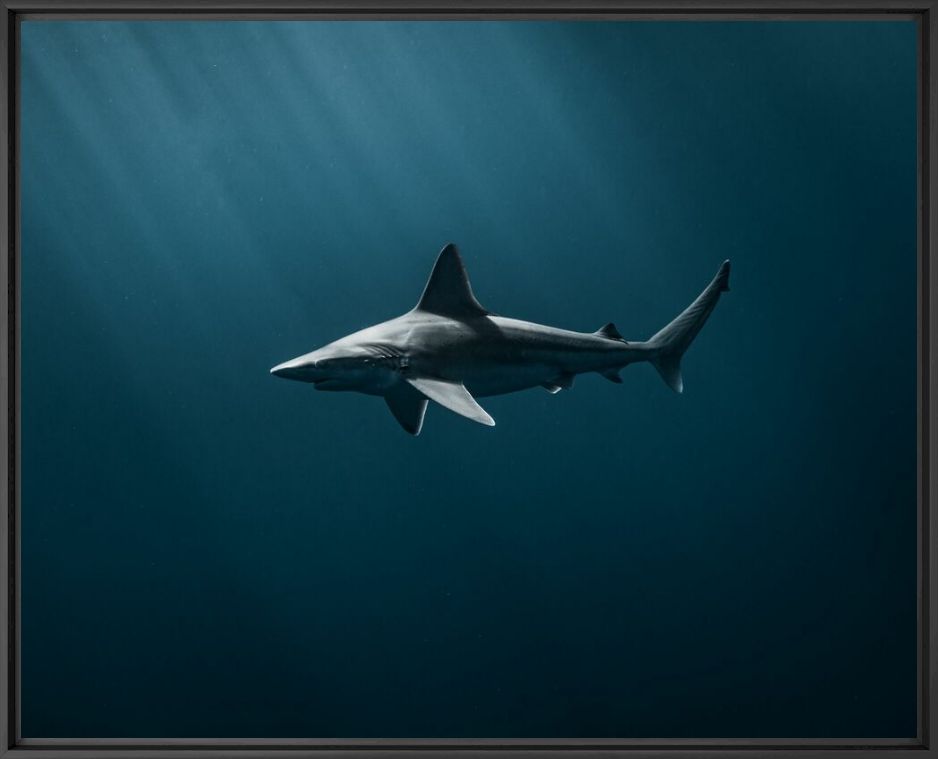The digital image captures a large gray shark swimming underwater, moving towards the left side of the frame. The shark's top is gray, while its belly is white. Both its fins are facing downwards. The water is predominantly dark and bluish-green, with a dramatic light source streaming from the top-left corner, casting rays diagonally towards the bottom right of the image. This light highlights the shark's snout, upper body, and left fin, giving them a brighter appearance. The shark is positioned centrally in the picture, surrounded by the medium blue to dark green hues of the water, which get darker towards the corners. The entire image is framed by a thin black and grey border, adding an additional sense of depth. The shark features a typical "shark grin," making it look both imposing and enigmatic.